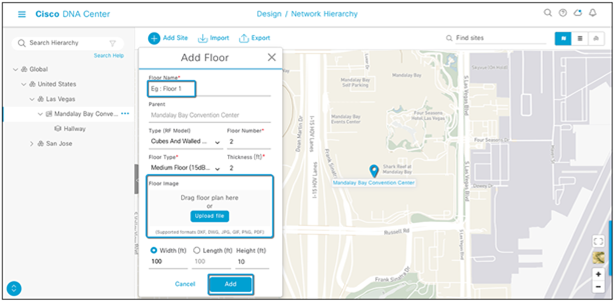The image features a user interface from the Cisco DNA Center Design Network. At the top, there is a white border displaying the title "Cisco DNA Center Design Network." Below the title, on the left side, is a search bar with some small, unreadable text beneath it. In the center of the image, a pop-up box labeled "Add Floor" appears, with a blue line underlining it. Under this header, there's an outlined blue text box, followed by an unreadable section of text and a blue rectangular button. 

Below this, another section of text is visible with one item highlighted and selected, indicated by a blue circular mark next to it. To the right of these items is another blue rectangular button. The right side of the image shows a map with a purplish tint, depicting several roads running vertically. There is a pin location marker and a zoom icon situated at the bottom right corner of the map.